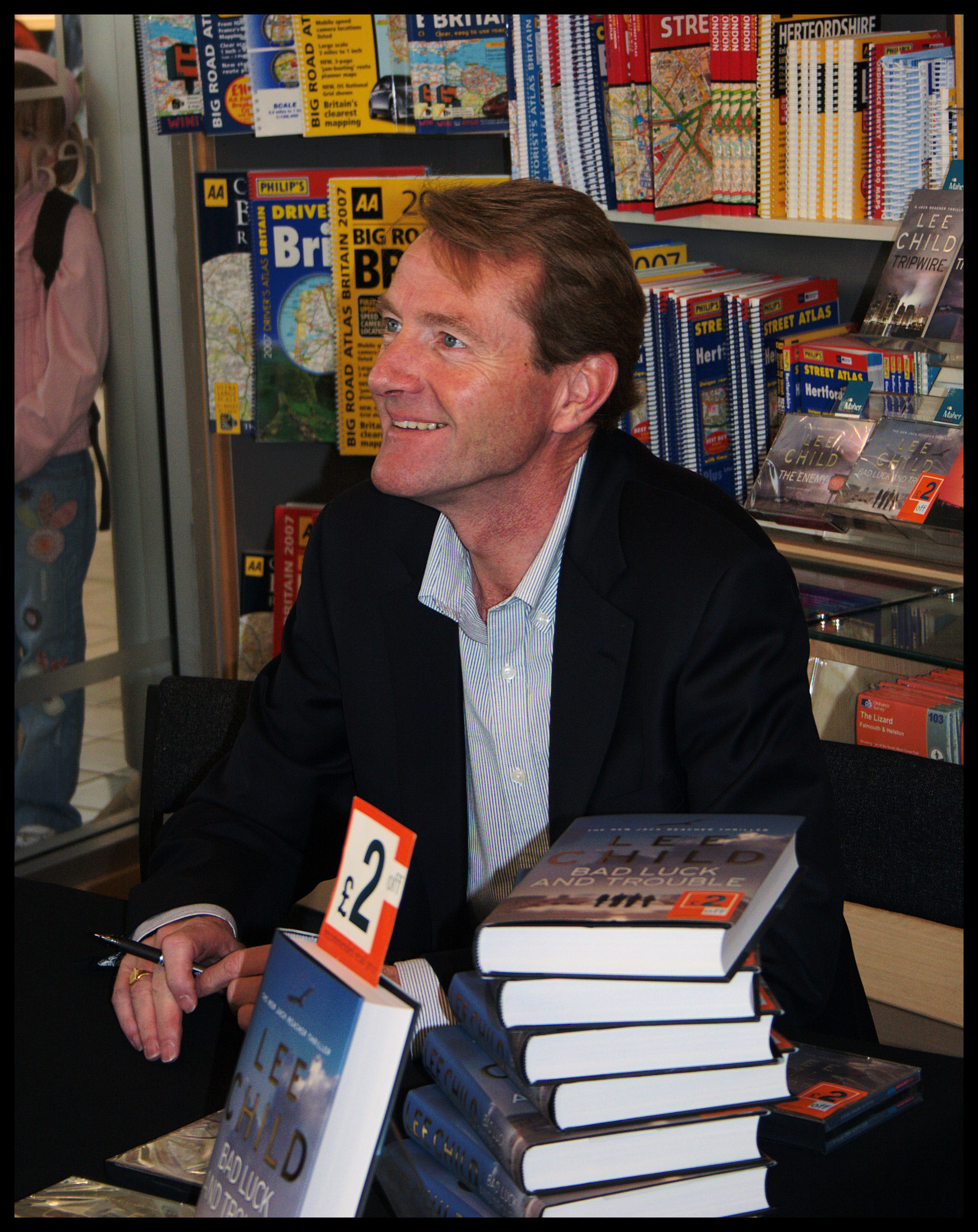The photograph captures a man, likely in his fifties, with darkish auburn hair and blue eyes, sitting at a table covered with a black tablecloth. He is dressed in a white and blue striped button-down shirt underneath a black blazer. The man is holding a black pen and smiling at someone off-camera to his left, suggesting he is engaged in a pleasant interaction. The setting appears to be a book signing event, as evidenced by the stacks of books on the table and the bookshelves filled with more books in the background. The books prominently display the title "Bad Luck and Trouble" and the author's name "Lee Child." In the upper left section of the image, partially visible through a window, is a little girl with a pink jacket, jeans with decorative flowers, and what looks like a backpack strap and a pink hat, observing from outside. The entire scene resembles a bookstore or a nice library ambiance.